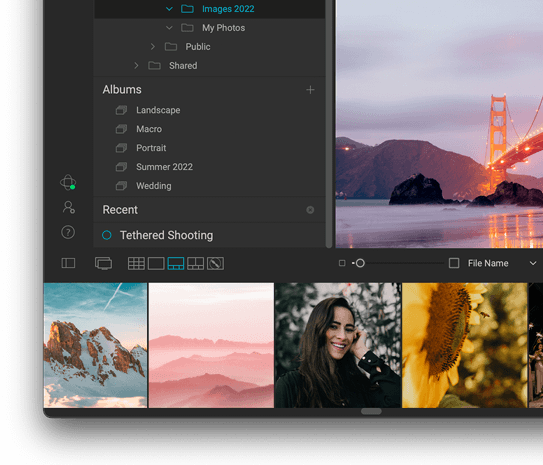The image depicts a partial view of a digital workspace that closely resembles Adobe Photoshop. The visible portion of the screen shows the file organization panel where multiple folders containing various images are displayed. Specifically, there are folders labeled "Landscape," "Macro," "Portrait," "Summer 2022," and "Wedding." 

To the right of this panel, the main workspace area features a striking photo of the Golden Gate Bridge set against a vibrant sunset. Additionally, there are several smaller thumbnail images visible: one shows majestic snowy mountains, another features a woman striking a pose, and yet another portrays mountains bathed in a pinkish hue, likely captured during dawn or dusk. The overall scene conveys a detailed and organized collection of diverse and captivating photographs.